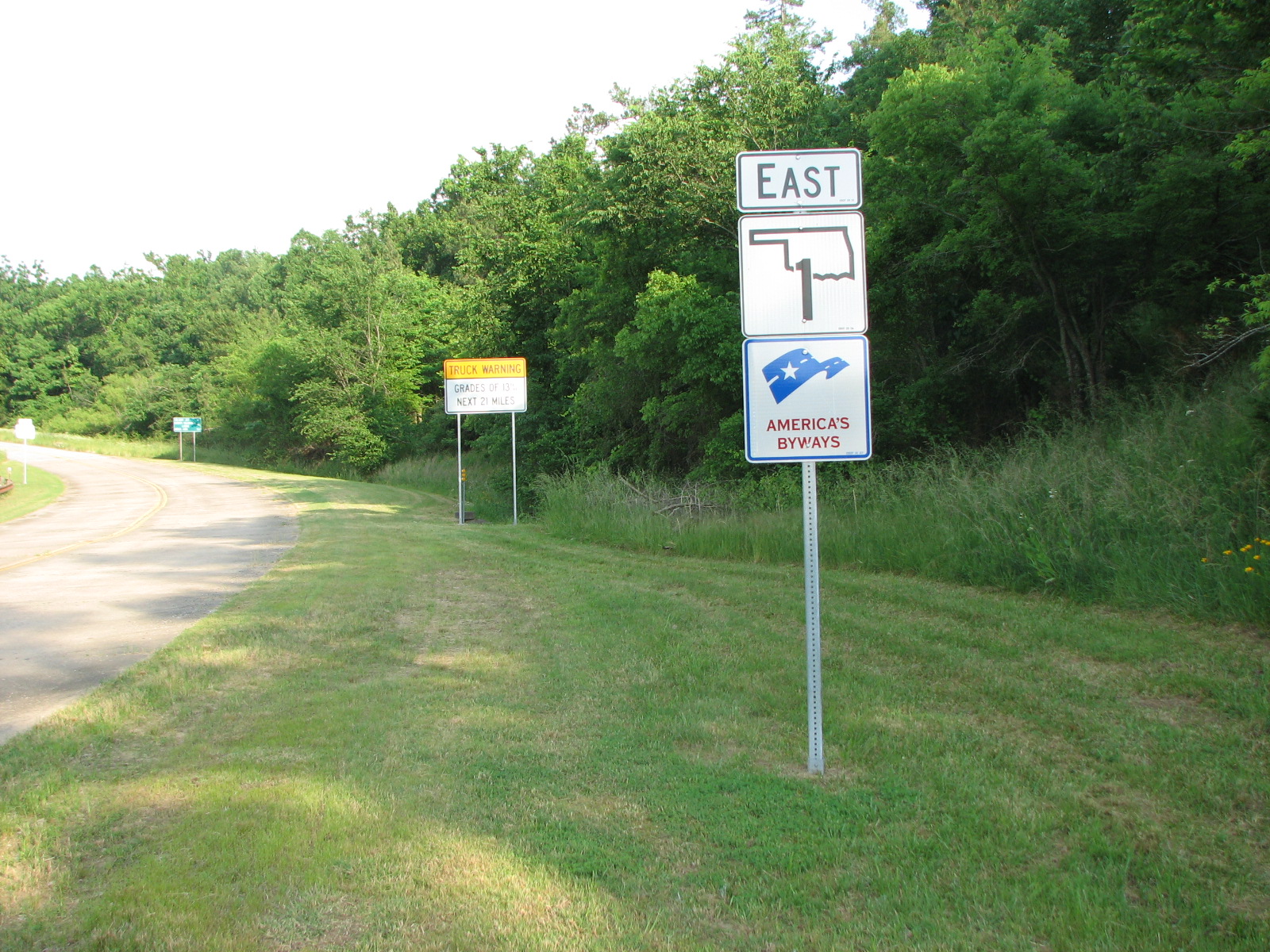A detailed photograph captures a scene on the side of a two-lane road, where a series of street signs are mounted on metal posts. The highway gradually curves to the left, with the photo taken from a vantage point about six or eight feet into the grassy area adjacent to the road. In the foreground, a sign prominently displays "East Oklahoma Highway 1" with an additional placard beneath it reading "America's Byways." A secondary sign situated just behind the first warns truck drivers of steep grades up ahead. The right side of the highway is flanked by lush greenery and dense trees, enhancing the natural, verdant backdrop.